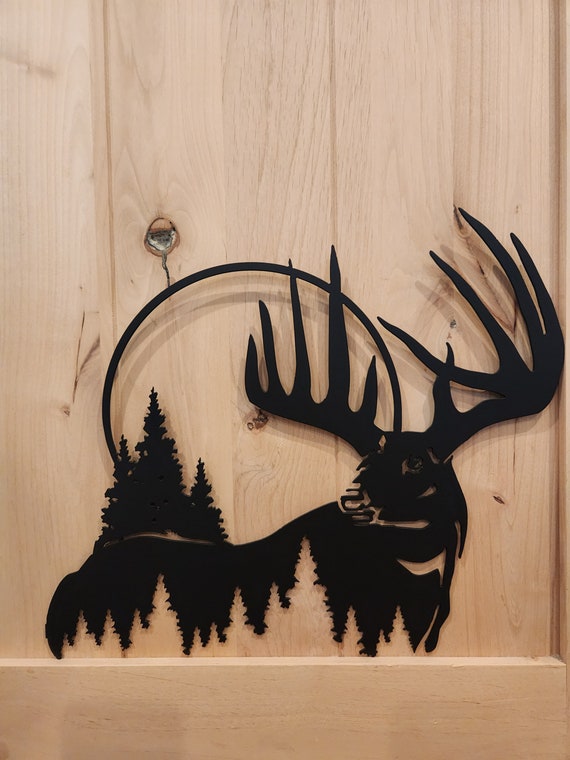The image showcases a detailed metal art piece, presumably laser-cut from a sheet of steel and painted black. The artwork features a large deer, or possibly an elk, with an impressive rack of antlers consisting of ten tines. The deer’s silhouette is intricately designed, incorporating the outlines of pine trees within its body. Behind the deer, additional trees and a circular shape resembling the moon are visible. The piece is mounted on a simple, light-colored wooden ledge, which appears to be made of pine plywood. Notably, there's a visible knot in the wood to the left of the photo. This artwork likely serves as a wall decor, ideal for a cabin or a home in a wooded area, potentially in the western United States where elk are commonly found.